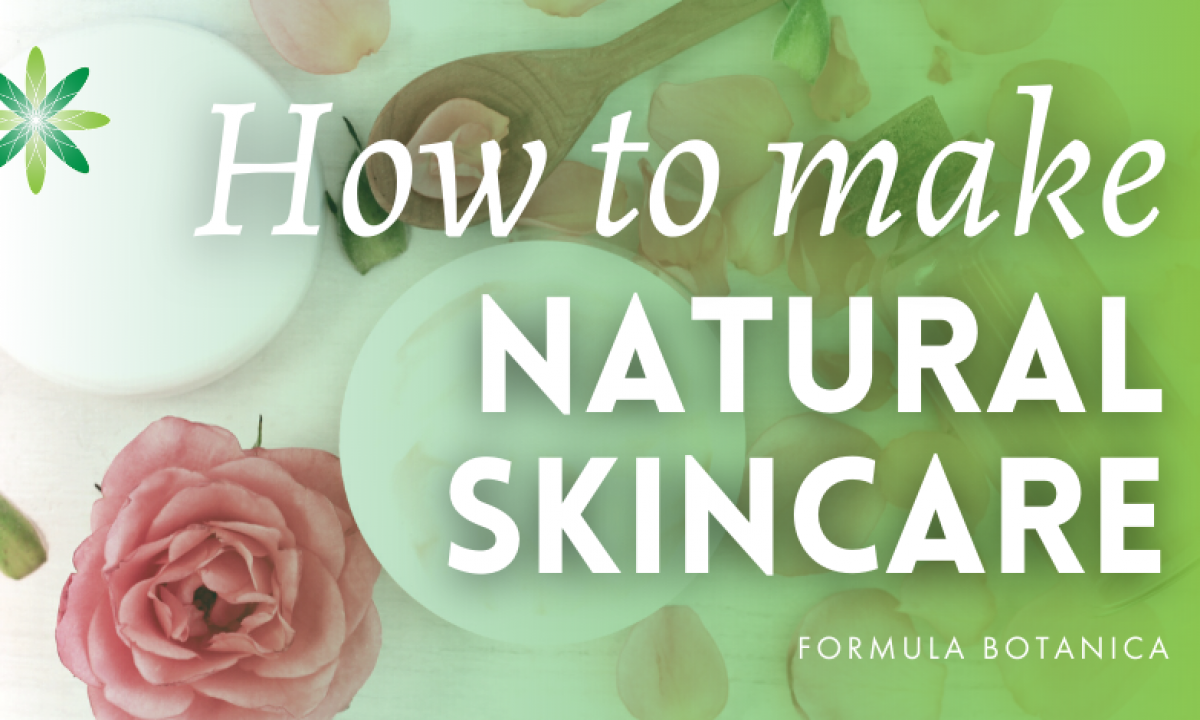The image appears to be the cover of an educational book or magazine on natural skincare. The design features a predominantly green background adorned with faint images of plants and leaves. In bold white text at the top, it reads "How to Make Natural Skin Care," while "Formula Botanica" is displayed in smaller white text at the bottom right corner. The layout includes a wooden spoon with a light pink flower petal at the top center, a green circle in the middle, and a white circle with light and dark green plants in the top left-hand corner. Additionally, there is a pink carnation flower in the bottom left-hand corner. The entire image is rectangular and horizontally oriented.